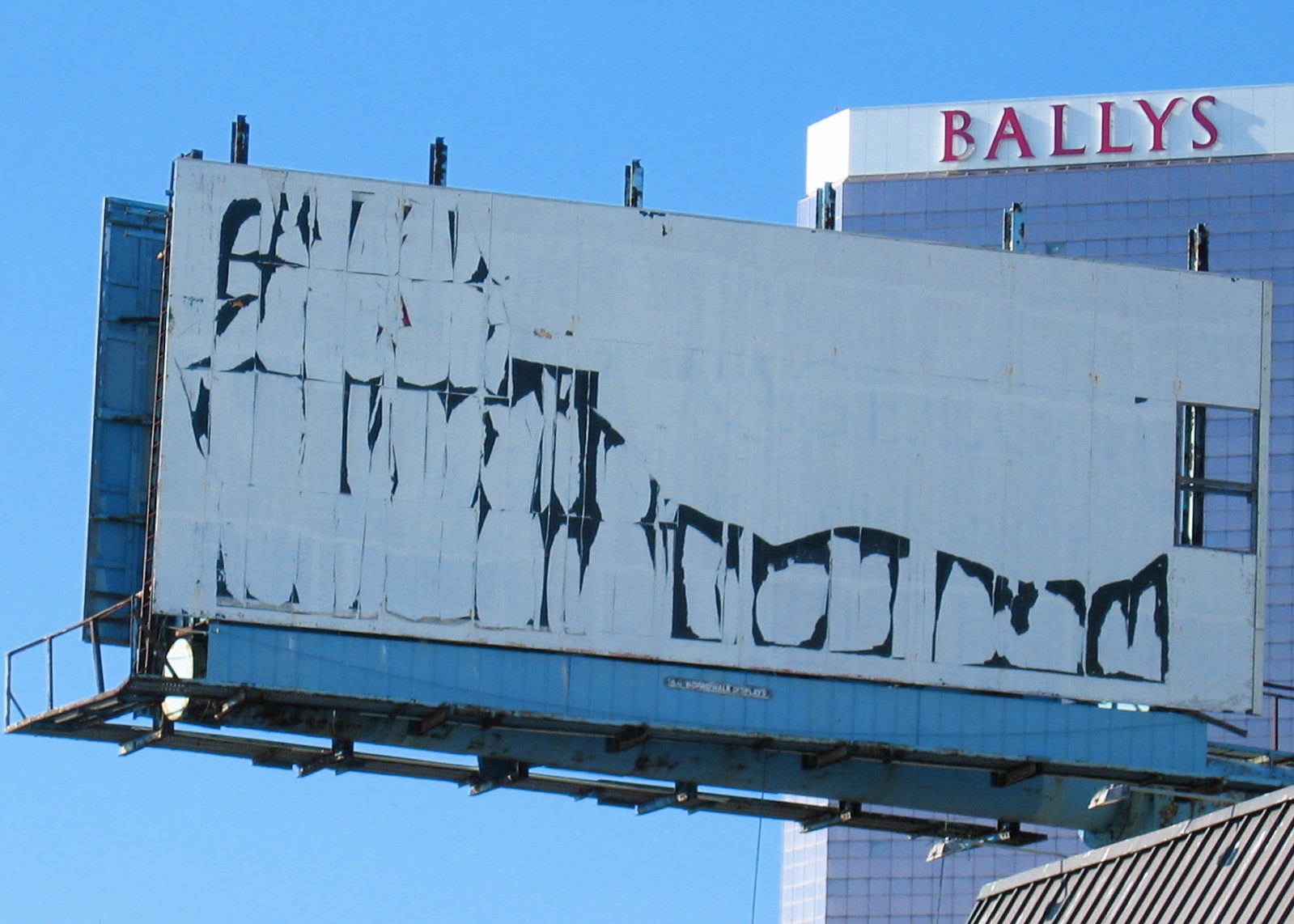This photograph captures an aging billboard that is visibly peeling, revealing patches of black beneath its deteriorating white paint. The right side of the billboard is missing several panels, allowing a clear view through to the structure behind it. The backdrop is dominated by a tall building, which could likely be an office or corporate headquarters. The building features the name "Bollies" written in red against a white section near the top. Below the sign, rows of windows extend from the nameplate down to the ground, giving the facade a sleek, modern appearance. The side of the building also has windows, but they appear in a lighter blue, almost white hue, contrasting with the blue-tinted windows on the front. The sky above is a vivid, uninterrupted blue, devoid of any clouds, further accentuating the structure and the worn billboard in the foreground.